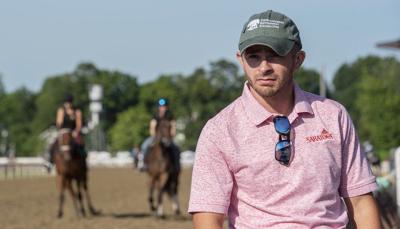The image is a full-color, rectangular photograph taken outdoors on a bright, sunny day with a completely clear blue sky. The background features a lush row of green trees that stretches horizontally across the image, suggesting late spring or summer. In the foreground, positioned on the right, is a man wearing a green baseball-style cap with white writing on it. He is dressed in a short-sleeve, pinkish-red collared shirt with writing on the left chest and sunglasses hanging from the collar. His arms are cut off at the upper arm by the edge of the image. Behind him, a wide dirt track can be seen, slightly blurred, with two riders on horseback—one on the left wearing something black and sleeveless, and one on the right wearing a green helmet. The track is bordered by a small white fence that encircles it. The blurry background consists of the row of trees, and above that, the vivid clear blue sky. The scene gives an impression that the man might be at a polo match or some other equestrian event, observing the horses and riders.